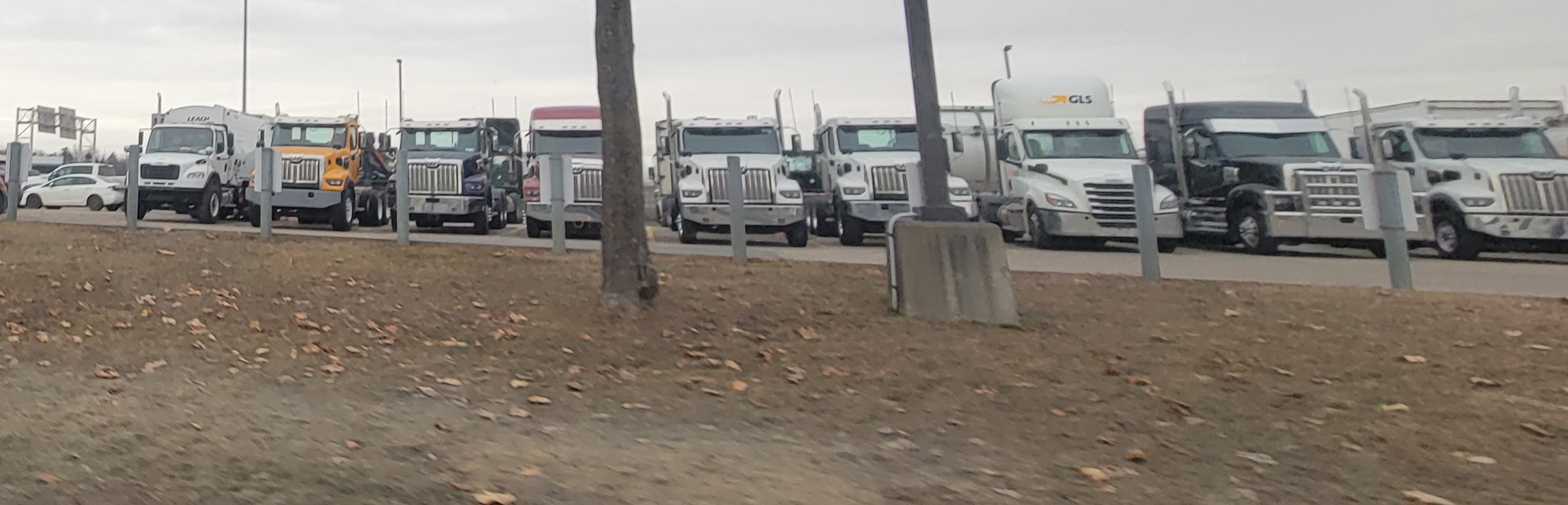The photograph captures an outdoor scene of a parking lot dedicated to tractor trailers and other trucks, taken on an overcast day. The central focus is on nine trucks aligned in a row, facing the camera with their cabs prominent. The trucks primarily consist of white cabs, with exceptions being a yellow truck and a black truck, all positioned behind a fence. Adjacent to the trucks, on the far left, a white car and a white pickup truck are also visible. The foreground of the image features a dirt area speckled with dried leaves, light posts, and what might be a tree trunk. Distant in the background, beyond the trucks, power lines and street lights are faintly noticeable, while the overcast sky looms above, casting a muted light over the scene.